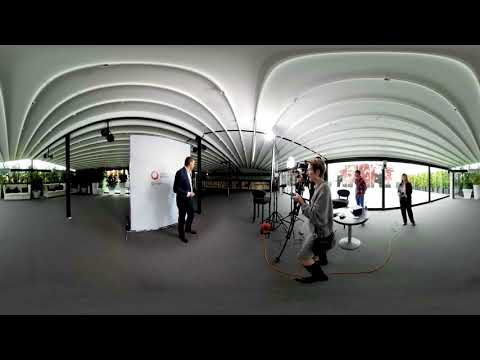The photograph captures an indoor setting resembling a tunnel or amphitheater with a unique white ceiling featuring a series of arching ribs. These arches create a symmetrical pattern reminiscent of ribs extending from both sides, and illuminate the central area. At the center of the composition, a photographer, equipped with a camera on a tripod and additional lighting, focuses on capturing an image of a man in a black tuxedo posing against a white backdrop adorned with a red symbol. The backdrop creates a professional photoshoot environment. Behind this setup, there are white couches accented with black pillows and well-maintained greenery visible, adding to the sophisticated atmosphere. The right side of the image reveals an expansive all-glass wall, through which bright daylight illuminates the interior, and outdoors, a line of meticulously trimmed bushes can be seen. Additionally, two individuals are busy near the glass wall, possibly writing on a table, further contributing to the busy yet organized ambiance. The dark gray carpeted floor accentuates the clean and modern aesthetic of the space.